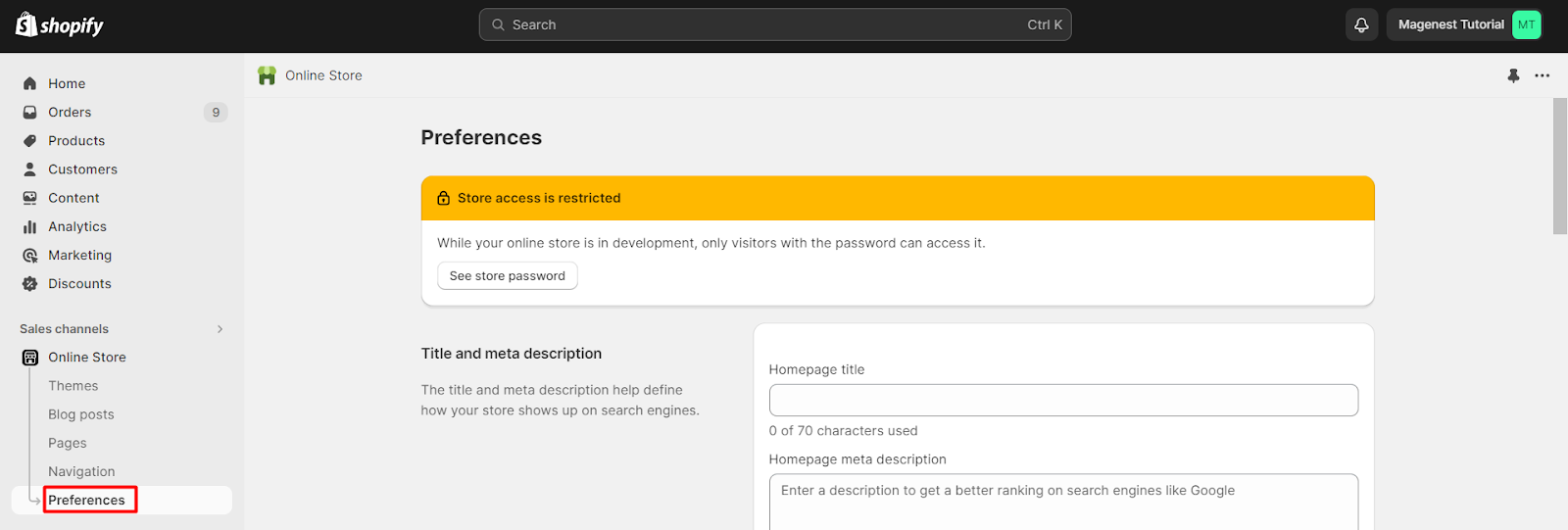A screenshot of a Shopify web page displayed on a laptop or PC. The interface, featuring a predominantly gray background with black lettering, is somewhat small, making it challenging to discern specific details clearly. At the top, a black banner with white text prominently displays "Shopify," along with a search bar for easy navigation. Below the banner on the left side is a vertical menu offering various navigational options: Home, Orders, Products, Customers, Content, Analytics, Marketing. To the right of this menu, another section titled "Online Store" appears, with a sub-option labeled "Preferences." This setup suggests that the user is likely configuring or managing their online store's settings and preferences within Shopify, customizing the website's appearance and functionality.